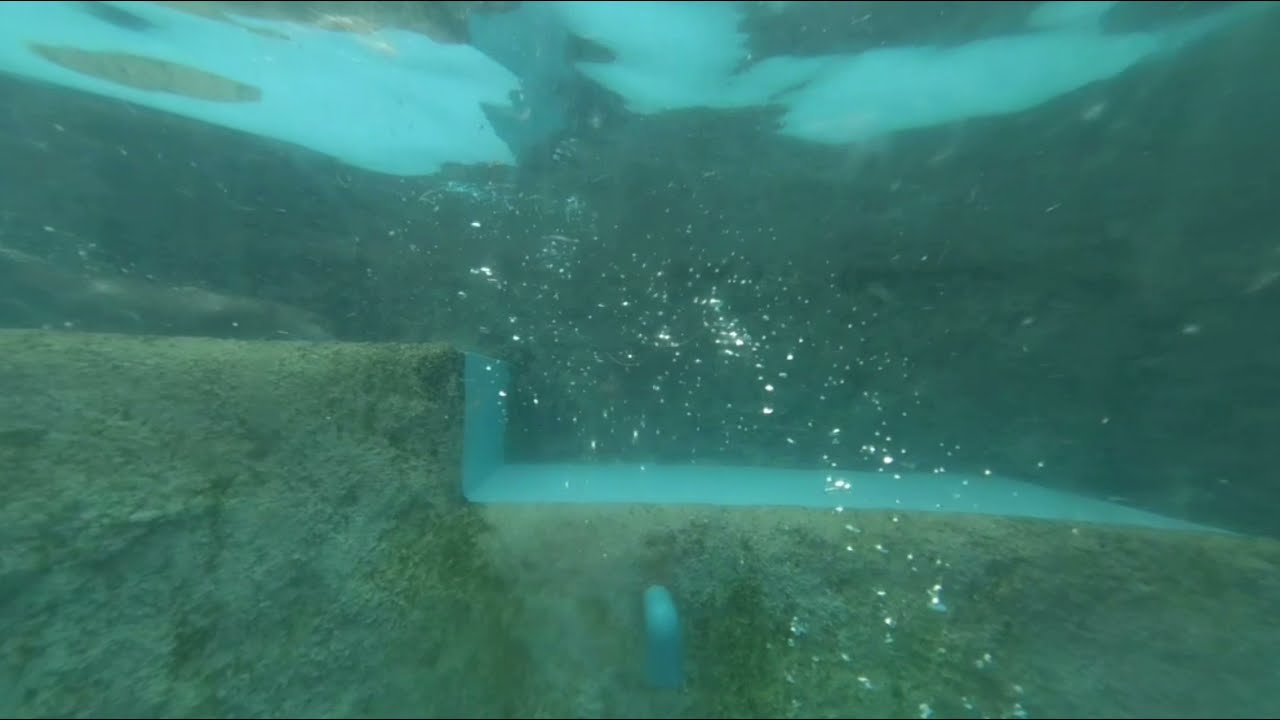This wide rectangular underwater image captures a detailed scene of a jagged, algae-covered surface resembling steps. Starting from the middle of the left edge, this surface progresses inward and downward like a step, showcasing a turquoise-hued top as it juts down and extends to the right. The gray sides of the steps are blanketed with green-gray algae, while the step surfaces are a clean, light blue, reminiscent of a pool. The photo appears to be taken about two to three feet underwater, highlighting a 90-degree inlet or outlet hose that matches the turquoise color of the steps. Bubbles cluster in the center, likely from the photographer, ascending through the brightly lit water towards a surface tinged with blue and dark green areas, suggestive of a daylight-lit environment without visible aquatic creatures. The underwater scene forms a vivid snapshot of an inviting, well-illuminated environment, reflecting a clear division of upper, middle, and bottom water layers.